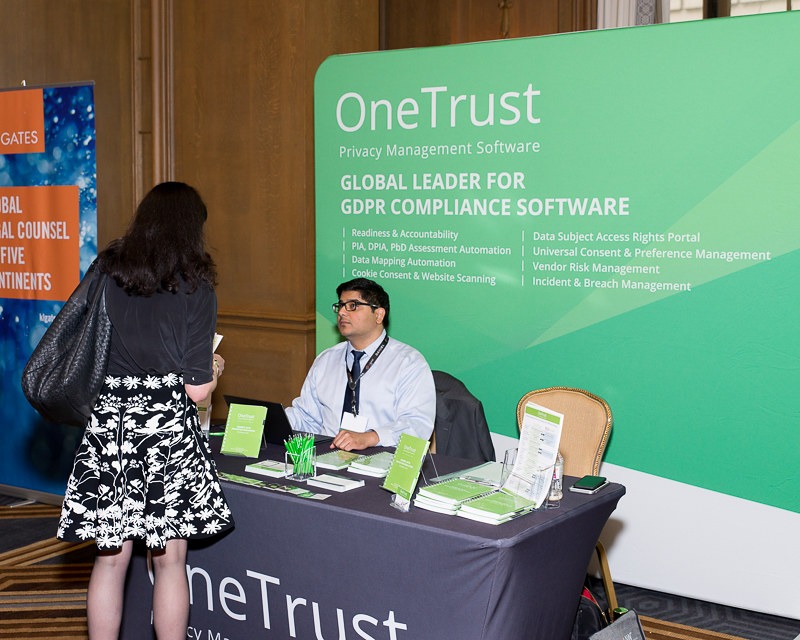The image captures a bustling scene at a job fair or trade show, with a focus on the OneTrust Privacy Management Software booth. Dominating the background is a large green sign that proclaims OneTrust as a "Global Leader for GDPR Compliance Software," highlighting key features like Readiness and Accountability, PIA, DPIA, Assessment Automation, Data Mapping Automation, Cookie Consent and Website Scanning, Data Subject Access Rights Portal, Universal Consent and Preference Management, Vendor Risk Management, and Incident and Breach Management. In the foreground, a young woman dressed in a black shirt and a black skirt adorned with white and yellow daisies stands facing a gentleman seated at the table, which is covered with a gray tablecloth featuring the OneTrust logo. She has a large black bag slung over her left shoulder and is holding a pamphlet, indicating she is likely gathering information about career opportunities or business services offered by OneTrust. The gentleman, who is seated in front of a laptop, is attentively engaging with her. To the left, another booth with blue and white signage featuring orange rectangles and white text can be partially seen, contributing to the vibrant atmosphere of the event.